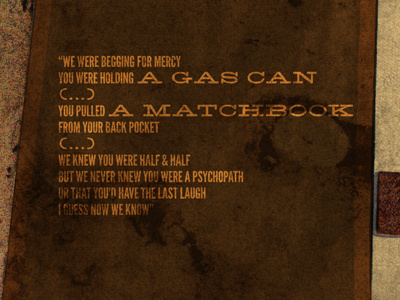The image features a wide vertical rectangular sign with a sandy-colored, possibly marble-like background. In the center, there is a slightly angled, dark brown wooden board or book cover, etched with a rustic, old-fashioned gold font in varying sizes. The prominent words "A Gas Can, A Matchbook" suggest this as the title. The text is written in all caps and reads: "WE WERE BEGGING FOR MERCY, YOU WERE HOLDING A GAS CAN... YOU PULLED A MATCHBOOK FROM YOUR BACK POCKET... WE KNEW YOU WERE HALF AND HALF, BUT WE NEVER KNEW YOU WERE A PSYCHOPATH, OR THAT YOU'D HAVE THE LAST LAUGH. I GUESS NOW WE KNOW." The poem within quotes portrays a dramatic and haunting scene, underscored by the worn, vintage aesthetic of the sign.